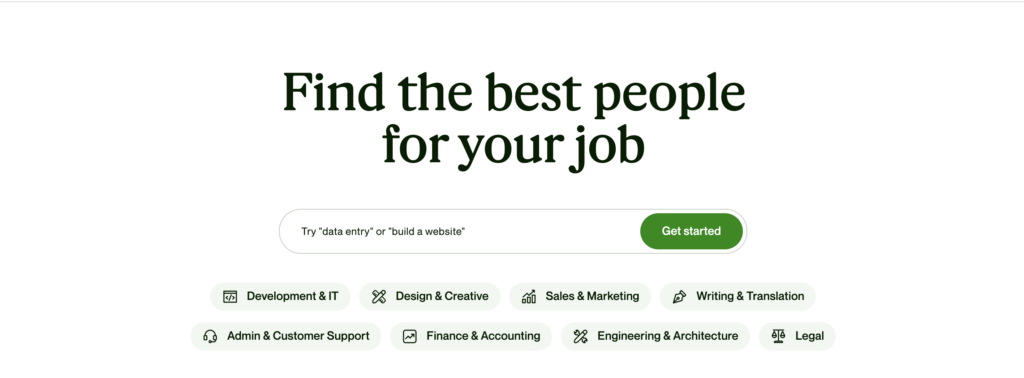The web page features a minimalist design with a pristine white background. A thin gray line stretches horizontally across the width of the page, creating a subtle visual break. About half an inch below this line, bold text declares, "Find the Best People," with a secondary, centered text beneath it reading, "For Your Job." Notably, only the first 'F' is capitalized while all other letters are lowercase.

Another half to a quarter inch below this section, a rounded rectangular white field juxtaposes with a green button to its right, labeled "Get Started" in white text. To the left of this button, in very small font, are the words, "Try Quotes, Data Entry, or Build a Website."

Further down, there's a row of navigation tabs. The first tab is labeled "Development and IT," followed by "Design and Creative," and then "Sales and Marketing."